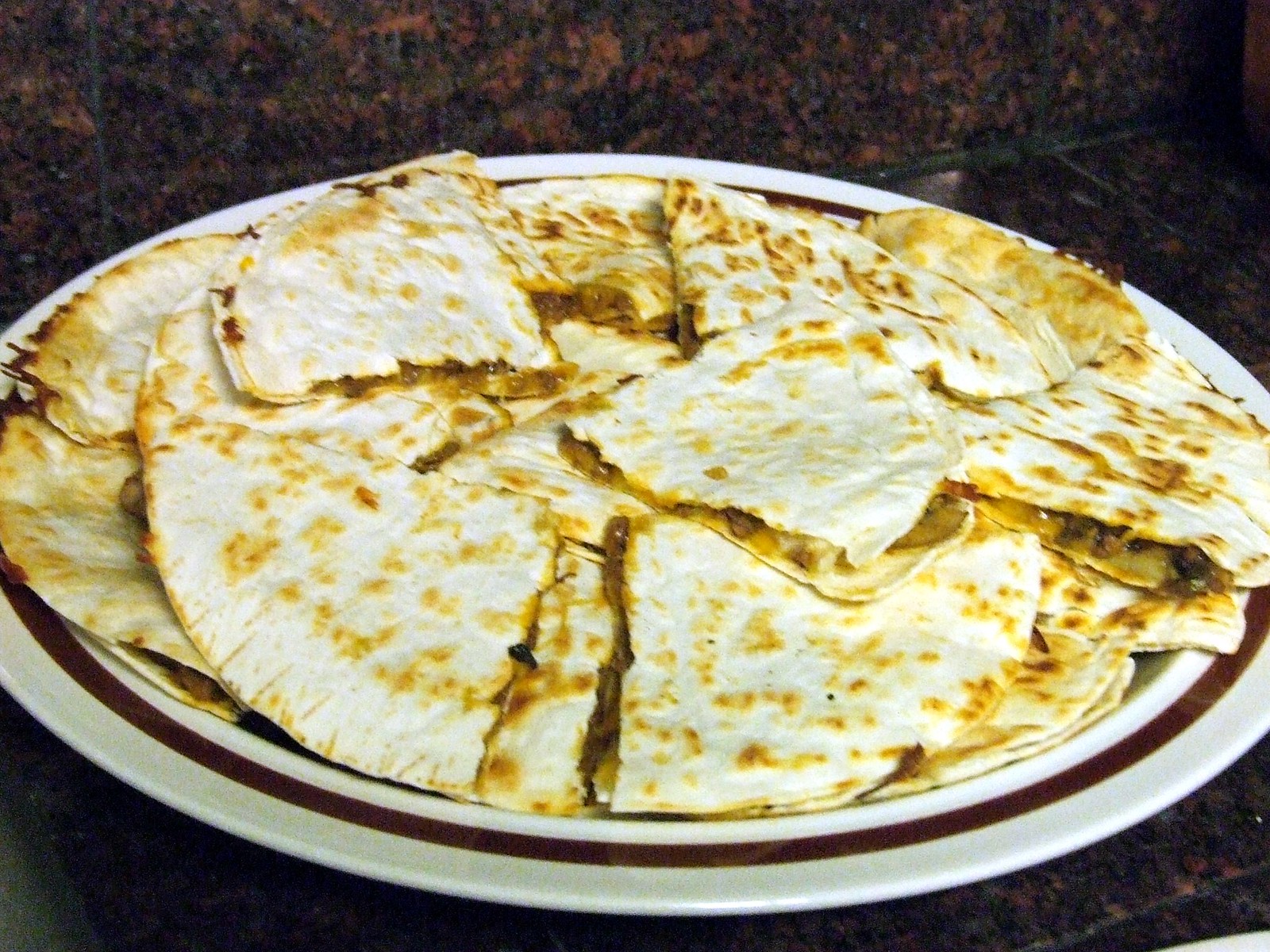The image displays a large number of toasted quesadillas neatly arranged on a circular white plate with a distinctive brown trim. The quesadillas, toasted to a golden brown with visible char marks, suggest the use of a grill. While the exact filling is not entirely clear, hints of dark meat or beans and possibly cheese are visible. This plate sits on a brown marbled granite tabletop, which continues into the matching backsplash in the background, creating a cohesive brownish-orange color palette throughout the photograph. The quesadillas and the detailed setting indicate significant effort and care in both the preparation and presentation.